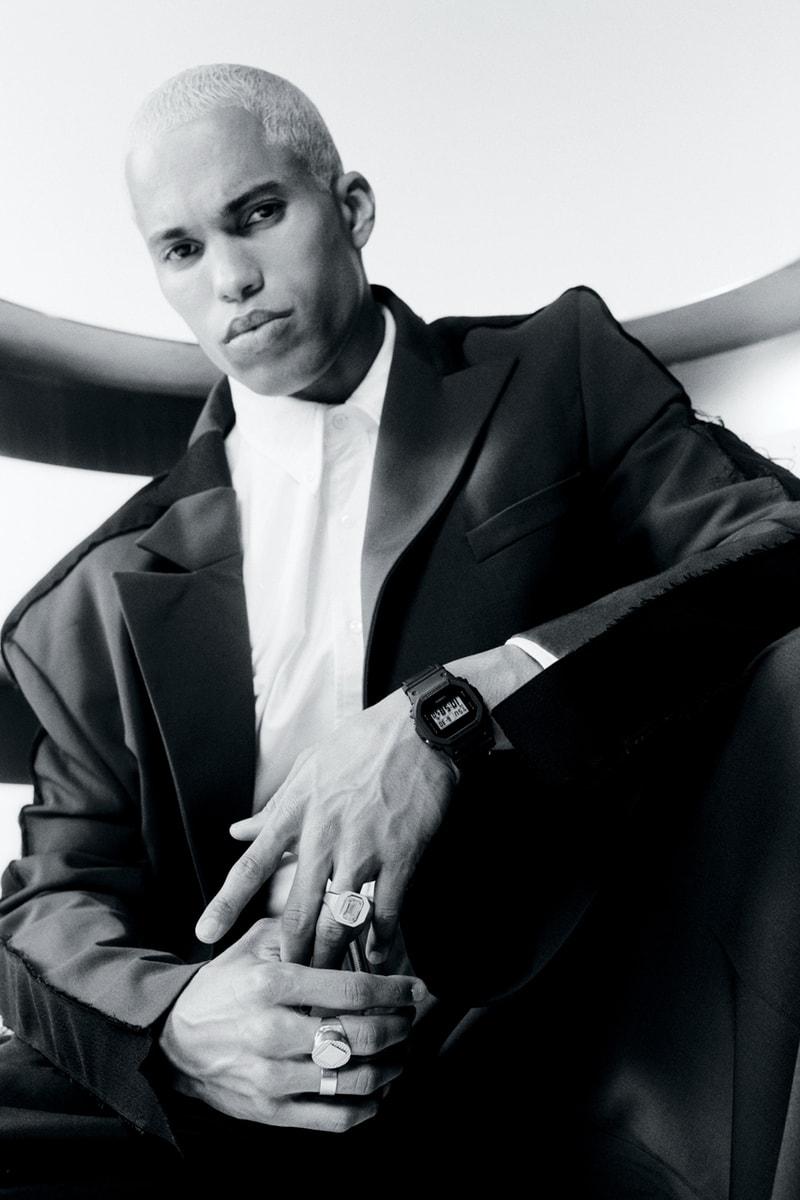The black and white photograph features an African-American man, likely in his late 20s or early 30s, exuding a confident and poised demeanor. His facial expression is serious, with lips slightly pouted and turned downwards, adding intensity to his gaze. The man has very short, bleached blonde hair that contrasts with his darker skin. He is adorned in an oversized black jacket that sits loosely on his thin frame, over a white button-up shirt. Large, possibly championship-style rings adorn his fingers, and he wears a simple black wristwatch. He is seated on a black chair, with his legs clad in black pants. The image, with its high-contrast grayscale tones, captures him looking down at the camera, suggesting a purposeful and stylized pose typical of modeling photography. The background is nondescript, only revealing the border of roof padding, keeping the focus entirely on the subject's striking appearance.